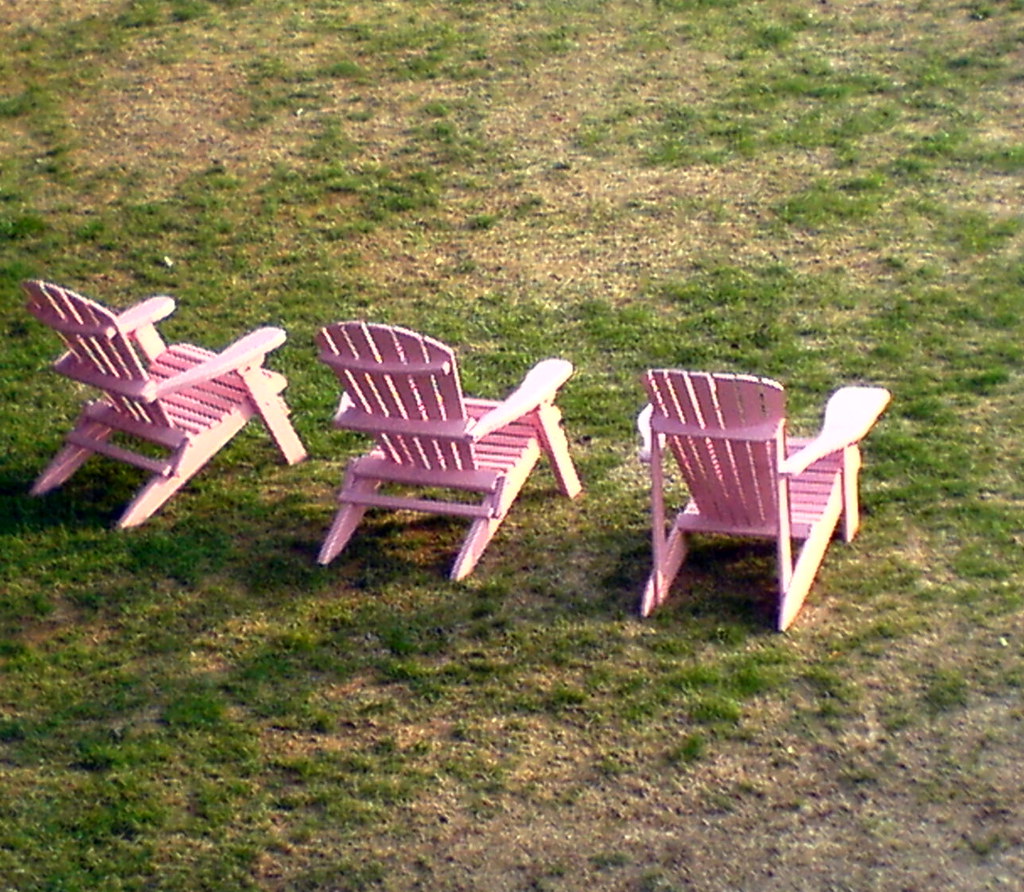This photograph captures three classic pink Adirondack chairs, also known as Muskoka chairs, made of wooden slats with horizontal seats and vertical backs, each equipped with armrests. They are arranged in a row facing away from the viewer, positioned on a slightly patchy, greenish-brown grassy field, suggesting early spring conditions or a lawn that has seen some wear and tear. The image, which is somewhat grainy and out of focus, appears to have been taken during an overcast day, though a gentle sunshine can be seen highlighting the chairs, casting their shadows off to the left and slightly behind. Despite the photo's less-than-perfect quality, it evokes a sense of relaxed outdoor leisure, with the chairs inviting viewers to sit back and enjoy the tranquility of the day.